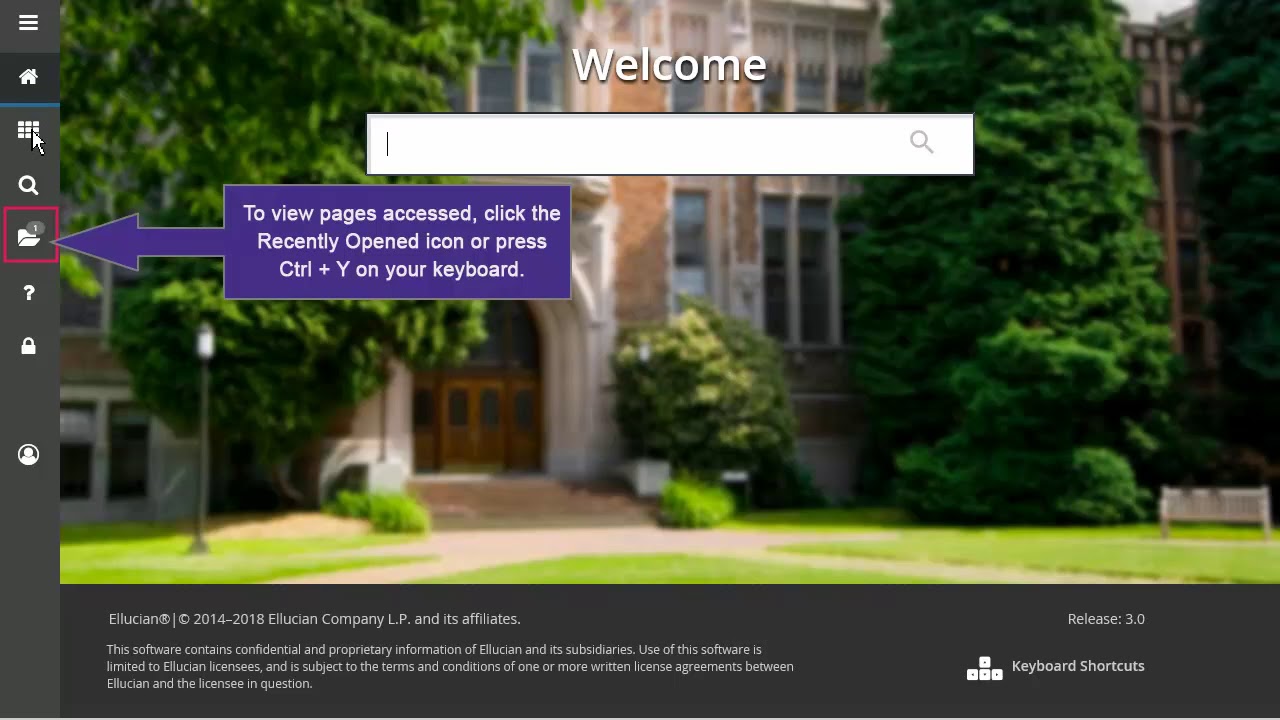In the screenshot, a slightly blurred background image of a building surrounded by large shrubbery on either side sets the stage. Overlaying the center of this image is the word "Welcome," with a search bar positioned directly below it. Along the left side of the screen, a vertical menu features several icons: a triple-line or "hamburger" menu at the top, followed by a home icon, a grid icon, and a search icon. Further down, there is a file icon encased in a red box. 

Overlaying the main building image, a purple box with an arrow provides instructional text: "To view pages accessed, click the recently opened icon or press Ctrl + Y on your keyboard." Below this informational overlay, there are additional icons, including a question mark, a padlock, and a profile icon, all in white and situated on a gray background strip. 

At the bottom of the screen, a similar gray strip houses small text containing a copyright date and some legal information. On the right-hand side of this lower strip, the text "Release 3.0" and "Keyboard Shortcuts" are visible.